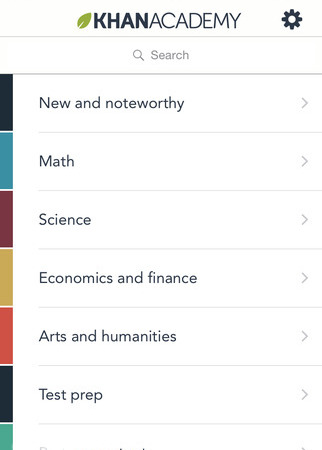This is a detailed and cleaned-up descriptive caption for the image:

"A cropped profile format screenshot from a smartphone, displaying the Khan Academy app. The Khan Academy logo, featuring bold text and a leaf emblem, is prominently displayed. Below the logo is a search function where users can type in topics to find relevant courses. The app’s interface also includes a menu bar with several colorful tabs for easy navigation. The tabs read 'New and Noteworthy,' 'Math,' 'Science,' 'Economics and Finance,' 'Arts and Humanities,' and 'Test Prep,' each highlighted in distinct colors: dark blue, light blue, maroon, light brown, light red, and dark blue respectively. The image does not display any specific phone features such as the name, time, or battery life."